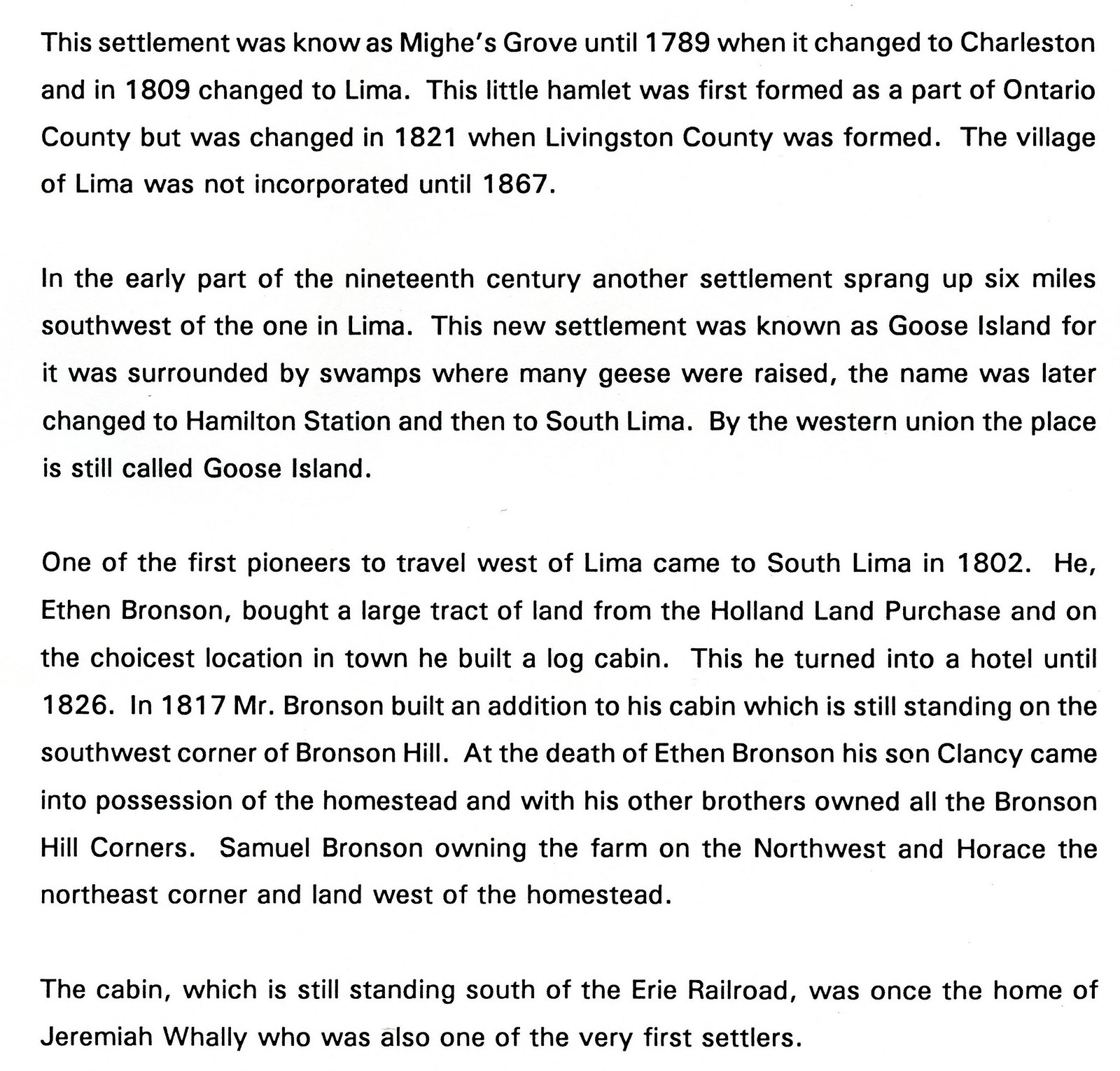The image is a screenshot from an educational website or email, featuring black text on a white background, formatted in a regular font. The text provides a detailed historical account of the settlement originally known as Ming's (or Meeks, Magus) Grove, which was renamed Charleston in 1789, and later Lima in 1809. Initially part of Ontario County, the hamlet became part of Livingston County upon its formation in 1821, but the village of Lima was not incorporated until 1867. Another settlement called Goose Island emerged in the early 19th century, located six miles southwest of Lima, later renamed Hamilton Station and then South Lima, but still informally known as Goose Island by the Western Union. Among the notable pioneers, Ethan Bronson established a log cabin in South Lima in 1802, which he operated as a hotel until 1826. The cabin he expanded in 1817 is still standing on Bronson Hill. Additionally, the text mentions a cabin south of the Erie Railroad, once home to early settler Jeremiah Wally.